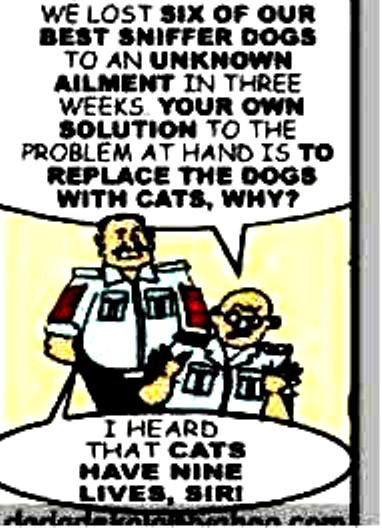This cartoon, reminiscent of a newspaper comic strip with noticeable pixelation, features a conversation between two characters set against a white backdrop with black and bolded text. The scene depicts a seated, bald man wearing a white shirt and circular glasses. He says, "We lost six of our best sniffer dogs to an unknown ailment in three weeks. Our own solution to the problem at hand is to replace the dogs with cats, why?" Standing next to him is a slightly chubby man with an official-looking mustache, also wearing a white button-up shirt that has red embellishments on the sleeves around the elbows. He responds, "I heard that cats have nine lives, sir."